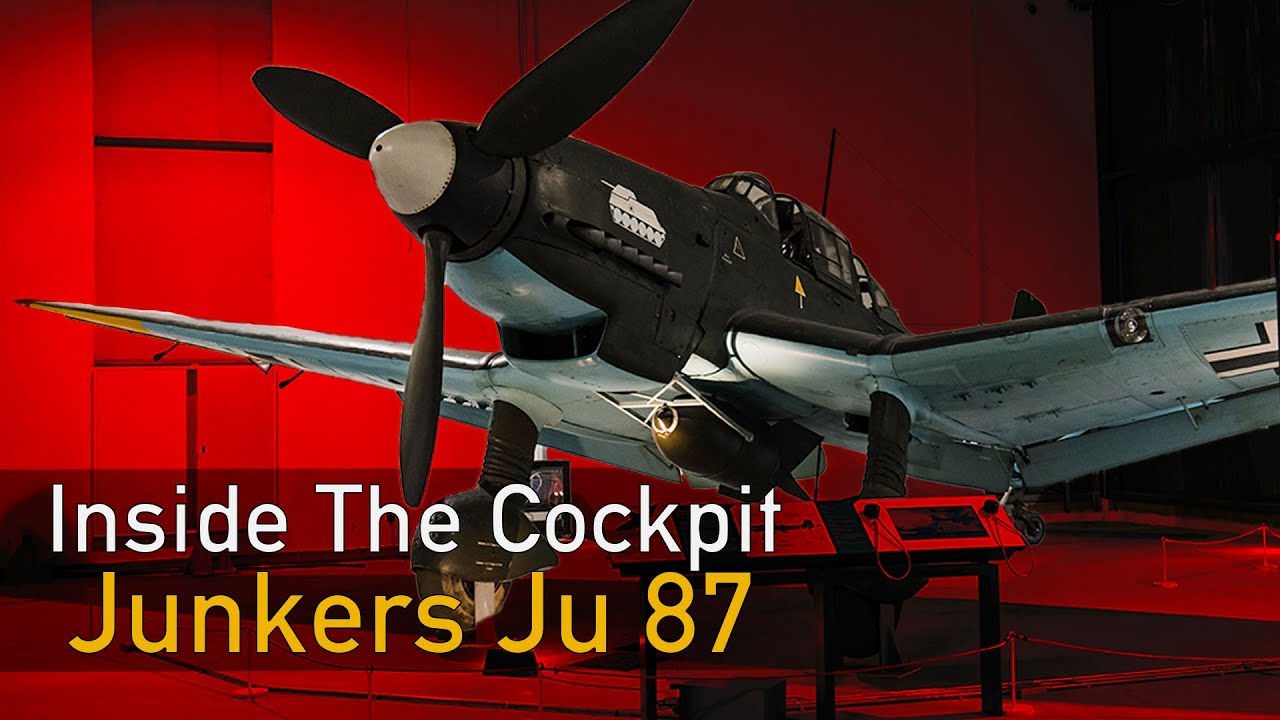This image features a computer-generated depiction of a vintage fighter jet, specifically a wartime Junkers JU-87, prominently displayed as if in a museum. The airplane, designed for a single pilot, is shown with a large propeller at the front, with black blades and white tips. The jet’s body is predominantly black, with a white tank painted on its top, while the underside of the wings and the belly of the plane are silver or light gray. A small, goldish bomb is attached beneath the plane.

The jet is slightly tilted upward, with its nose pointing to the left and up, adding to its aggressive stance. The backdrop of the scene transitions from a vibrant red on the left, potentially highlighted by a light source, to a darker, shadowed red on the right. The ground, also red, has roping around the jet to indicate it cannot be approached closely, reinforcing the museum-like setting. On the bottom left, white and yellow lettering reads “Inside the Cockpit, Junkers JU-87.” The image exudes a sense of historical reverence and showcases the aircraft against the striking red and black background.